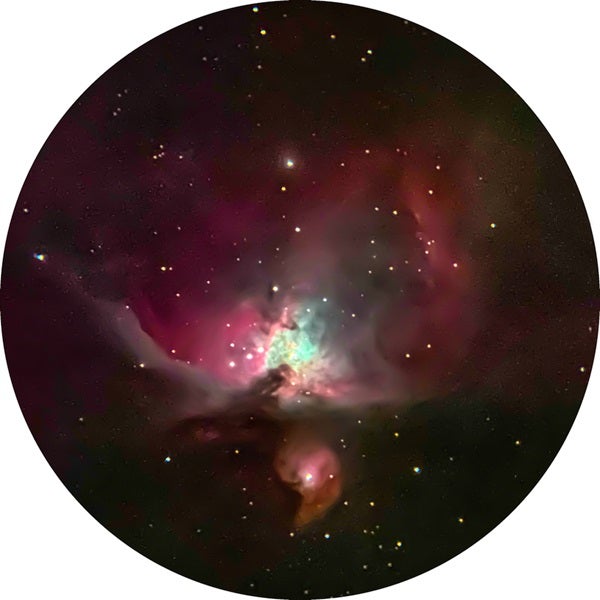The circular image presents a mesmerizing and sci-fi-esque depiction of the universe, rich with deep and intense colors. At its center, a brilliant bluish-yellow-green light bursts forth, creating a vivid focal point amidst the celestial scene. Surrounding this central light, a cloud-like, gaseous nebula in shades of purple, pink, and red spirals outward, interspersed with darker hues of brown and black. This nebula dominates the space, adding a textured, almost magical quality to the image. Numerous bright, shiny stars, appearing as small balls of white and yellow, dot the composition, contrasting against the pervasive blackness of space that frames the scene, particularly toward the perimeter. Beneath the central light, thicker, dark swirls resembling clumps of dust and shadows add depth and complexity, contributing to the overall mystical atmosphere of the image.